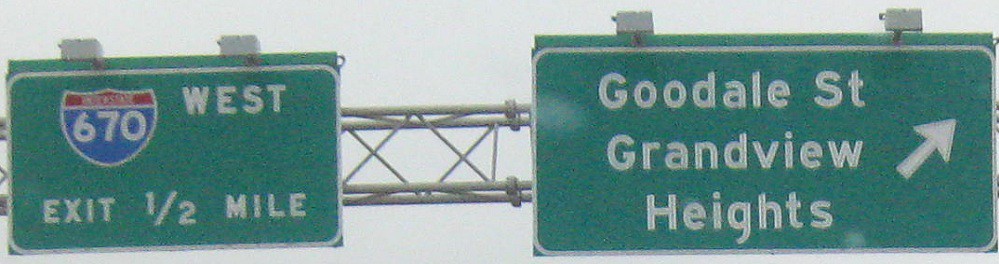This photograph depicts two green highway directional signs mounted on a metal brace extending over a roadway on the east coast of the United States. The left sign, embossed with an Interstate 670 shield in red, white, and blue, reads "670 West, exit 1/2 mile." To the right is a rectangular sign with larger white lettering that says "Goodale Street, Grandview Heights," accompanied by an upward and right-pointing arrow. Both signs feature white writing on a green background with white pinstriping around the edges. They are flanked by floodlights—two on each sign. The signs are set against a backdrop of a cloudy, overcast sky, with visible gray scaffolding. The roadway itself is not visible in this image.